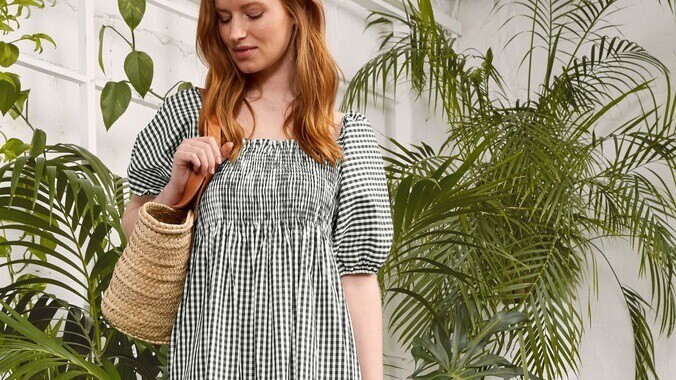In this detailed photograph, a red-haired young woman stands against a white, industrial-style wall, suggesting a converted building space. She is clad in a black and white gingham summer dress, featuring poofy elbow-length sleeves, a square neckline, and a smocked, shirred bust that extends into a high empire waist. Her red hair flows past her shoulders, and she carries a woven straw shoulder bag over her right shoulder, her hand grasping the handle. Her eyes are downcast with a partial smile, giving a sense of serene introspection. Positioned slightly to the left of center in the photo, she is framed by an array of lush house plants, including sizable ferns and hanging pothos, along with palm trees that add vibrant greenery to the scene. The background is stark white, possibly a window with shades drawn, enhancing the crisp, clean aesthetic of what could be a fashion photo shoot.